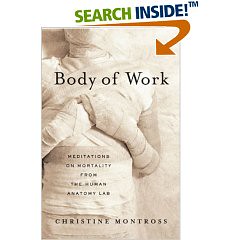This image appears to be an online book advertisement, likely from a website like Amazon. It features the cover of a book titled "Body of Work: Meditations on Mortality from the Human Anatomy Lab" by Christine Montross. The cover depicts a top-down image of a woman lying on a bed, wrapped entirely in white bandages, resembling a mummified state. The image is focused from her chin down to her pelvis, with her arms and hands positioned across her chest, suggesting a death-like posture. At the top of the image, there is an arrow labeled "Search Inside TM" which hints at the interactive feature to preview the book's contents. This visual metaphor suggests themes of mortality and the body’s condition after death, aligning with the book's exploration of human anatomy and life's transient nature.